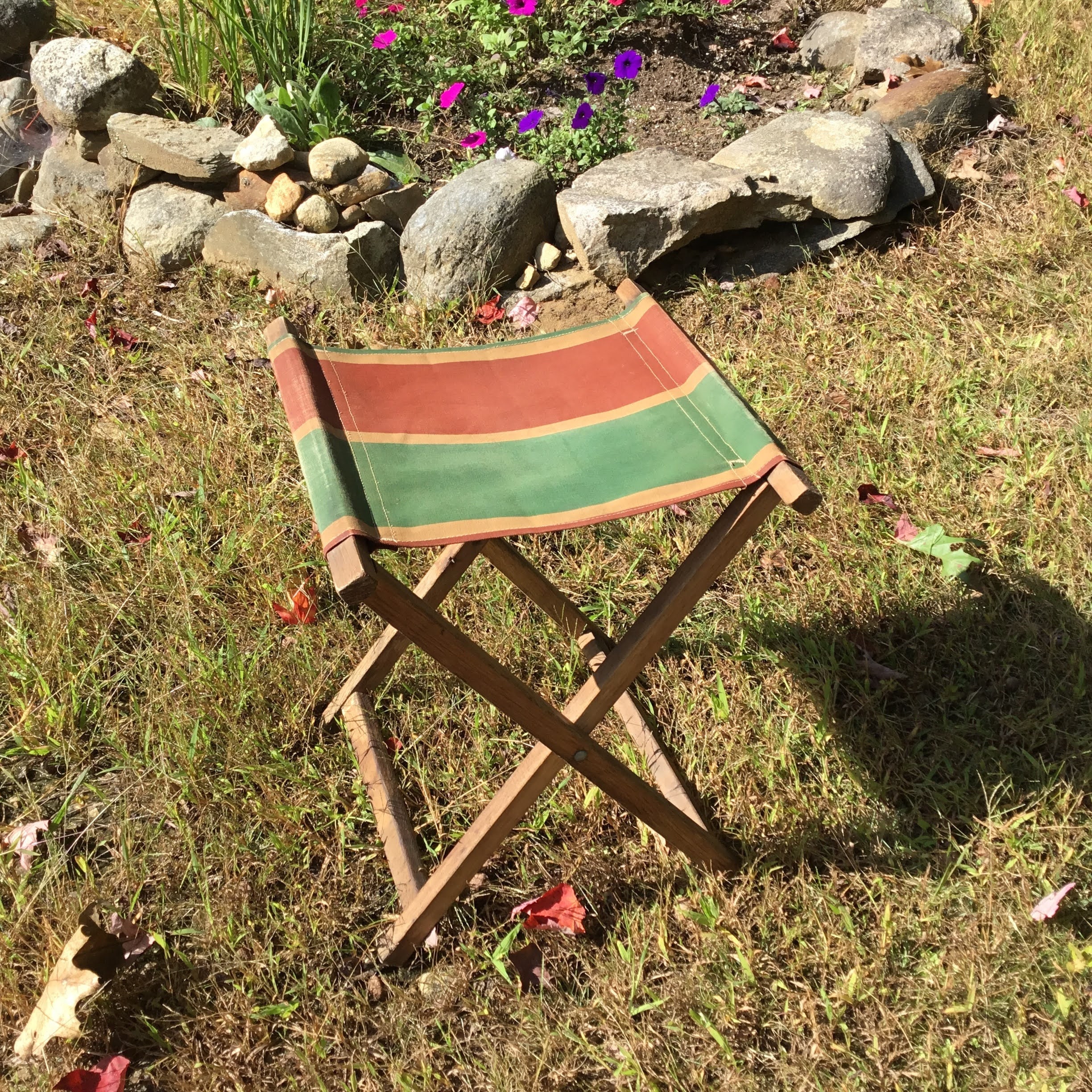In this outdoor photograph, the scene is centered around a foldable wooden stool featuring a seat crafted from a tapestry with orange-yellow stripes across sections of reddish-orange and green colors. Positioned on a patch of dried, brown grass interspersed with scattered red and green leaves, the stool's base forms an X shape typical of filmmaker chairs. Above the stool, at the upper edge of the image, a garden bordered by large rocks is visible. This garden showcases diverse vegetation, with green plants emerging from the soil and vibrant magenta and purple flowers in full bloom.